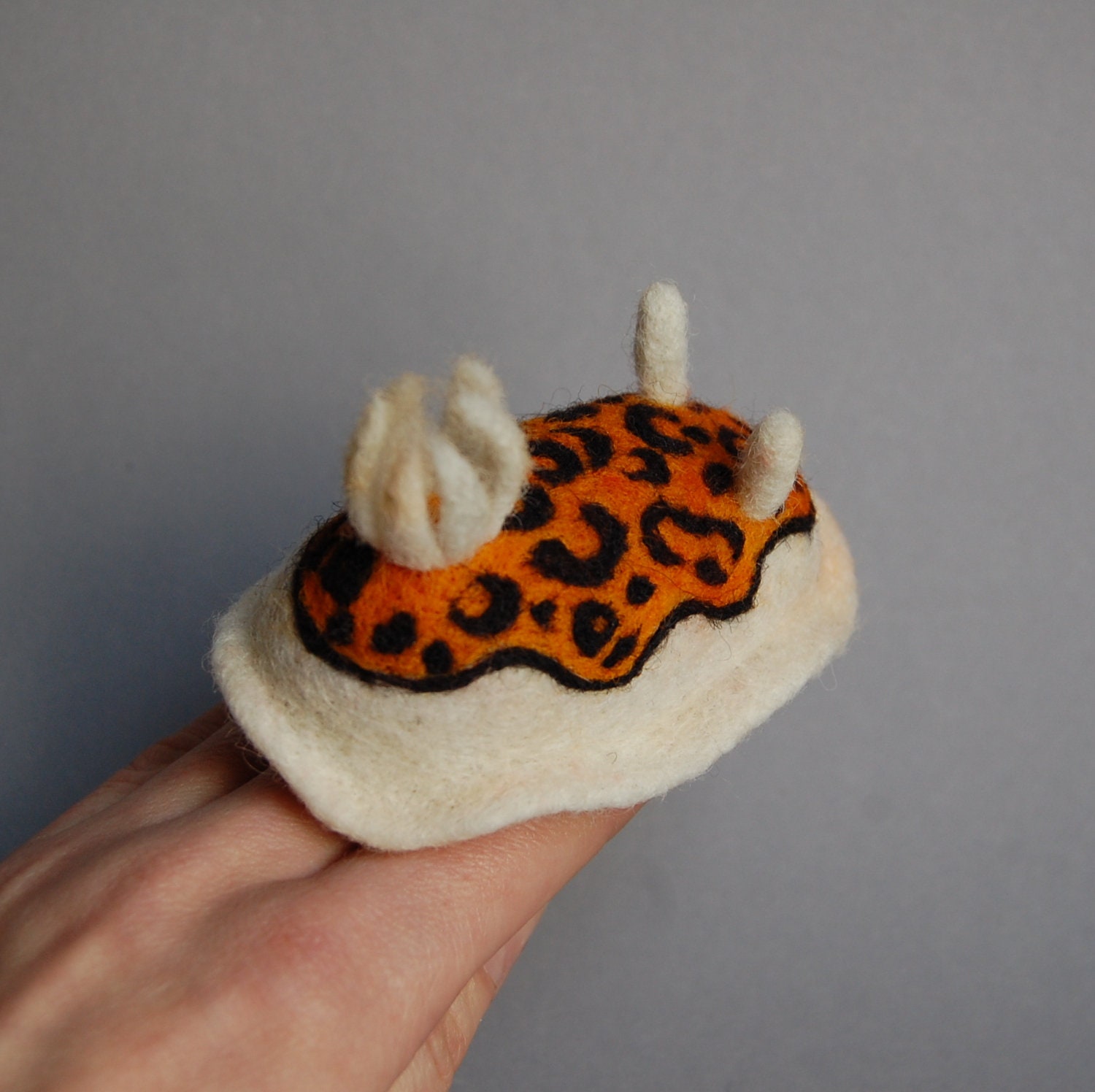The image is a vertical rectangular photograph showcasing a person's left hand extending from the lower left corner towards the center of the frame. The back of the hand is visible with the fingers together, providing a platform for a small handcrafted object made of clay. The object, resembling a whimsical bug or slug, sits atop the fingers. It is oval-shaped with two antennae protruding from the top, painted primarily orange with a black edge outlining the orange. The interior section features black semicircles and dots scattered artistically, complemented by a small white detail that resembles an opening flower. The background is a light gray wall, slightly dim, adding a soft, neutral backdrop to highlight the hand and the unique clay creation. The handcrafted object is exquisite, bearing a look similar to a stuffed toy with a leopard print-like pattern and fuzzy white accents, potentially offering the illusion of a cozy warmer when placed on fingers.